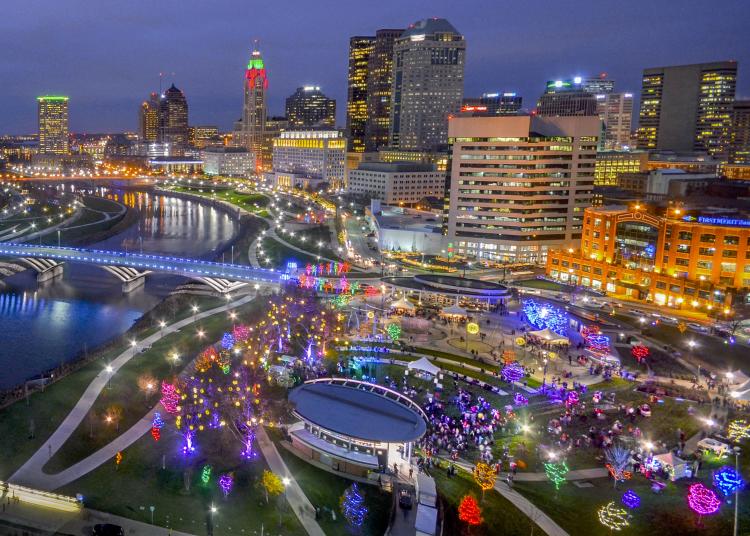This aerial photograph, likely captured by a drone or airplane, showcases a vibrant nighttime cityscape dominated by a well-lit urban park. The dark blue sky of the scene strongly indicates that the photo was taken at night. A bustling metropolis emerges in the background with numerous skyscrapers and multi-story buildings, their interiors and rooftops illuminated, casting a luminous glow over the skyline. These structures vary in color, shape, and size, adding a dynamic visual interest to the horizon.

On the left side of the image, a river curves gracefully into the city, spanned by a large bridge supported by multiple gray columns. The bridge itself and its surroundings are adorned with white LED lights, enhancing its prominence within the scene. 

The park, occupying the bottom half of the photo, is a lively, festive space. It features numerous pedestrian walkways paved in white cement, frequented by people. The park's trees, despite being bare of leaves, are festooned with dazzling LED lights in vibrant colors like pink, blue, green, and yellow. This array of colorful lights suggests a celebratory atmosphere, perhaps a festival or seasonal event. 

The overall image, brimming with lights and activity, captures the harmonious blend of urban development and communal recreational space, epitomizing the city's nighttime energy and charm.